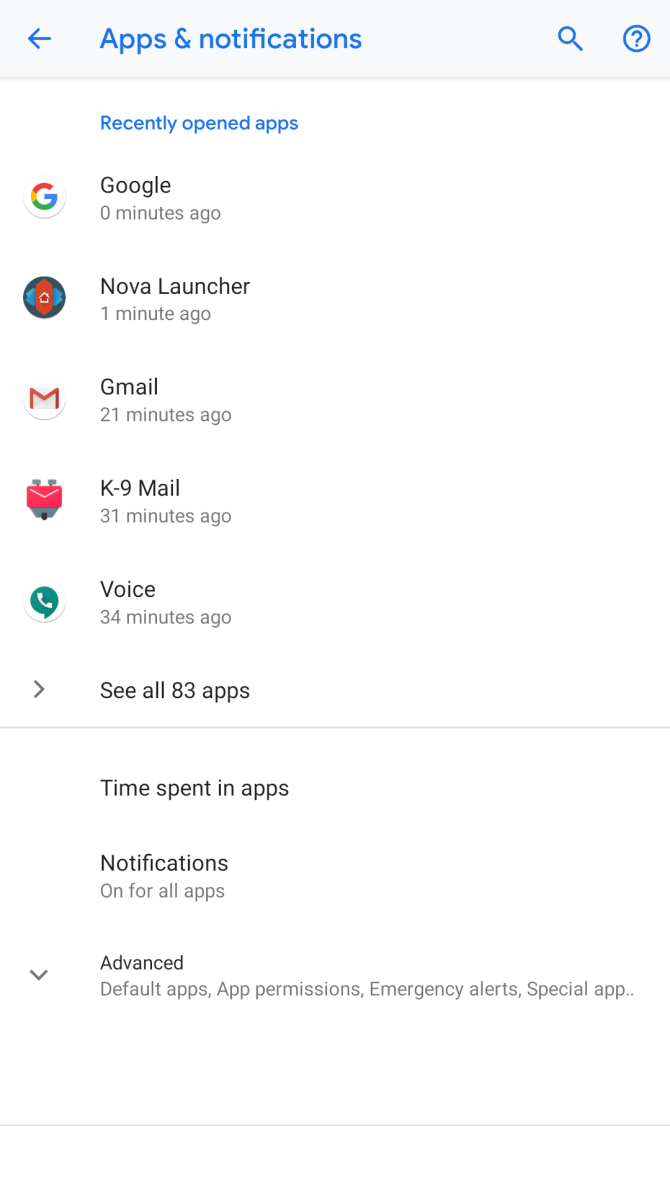The image depicts a screenshot of the "Apps and Notifications" settings screen. At the top of the screen, there is a title in blue text that reads "Apps & notifications." On the left side of the header, a left-pointing arrow is visible, while the right side of the header features a magnifying glass icon and a circle with a cross mark inside it. The header is set against a light gray background.

Below the header, the section titled "Recently opened apps" appears in blue text. Underneath this heading, a list of recently accessed apps is displayed in the following order:
1. Google - 0 minutes ago
2. Nova Launcher - 1 minute ago
3. Gmail - 21 minutes ago
4. K9 Mail - 31 minutes ago
5. Voice - 34 minutes ago

At the bottom of this list, there is an option to "See all 83 apps."

Further down, the screen shows additional sections including "Time spent in apps," "Notifications," and "Advanced," which offers further settings like default apps, app permissions, emergency alerts, and special app access.

The main background of the image is white, with the exception of the light gray strip at the top. The design and layout are clean and organized, ensuring easy navigation through app-related settings.